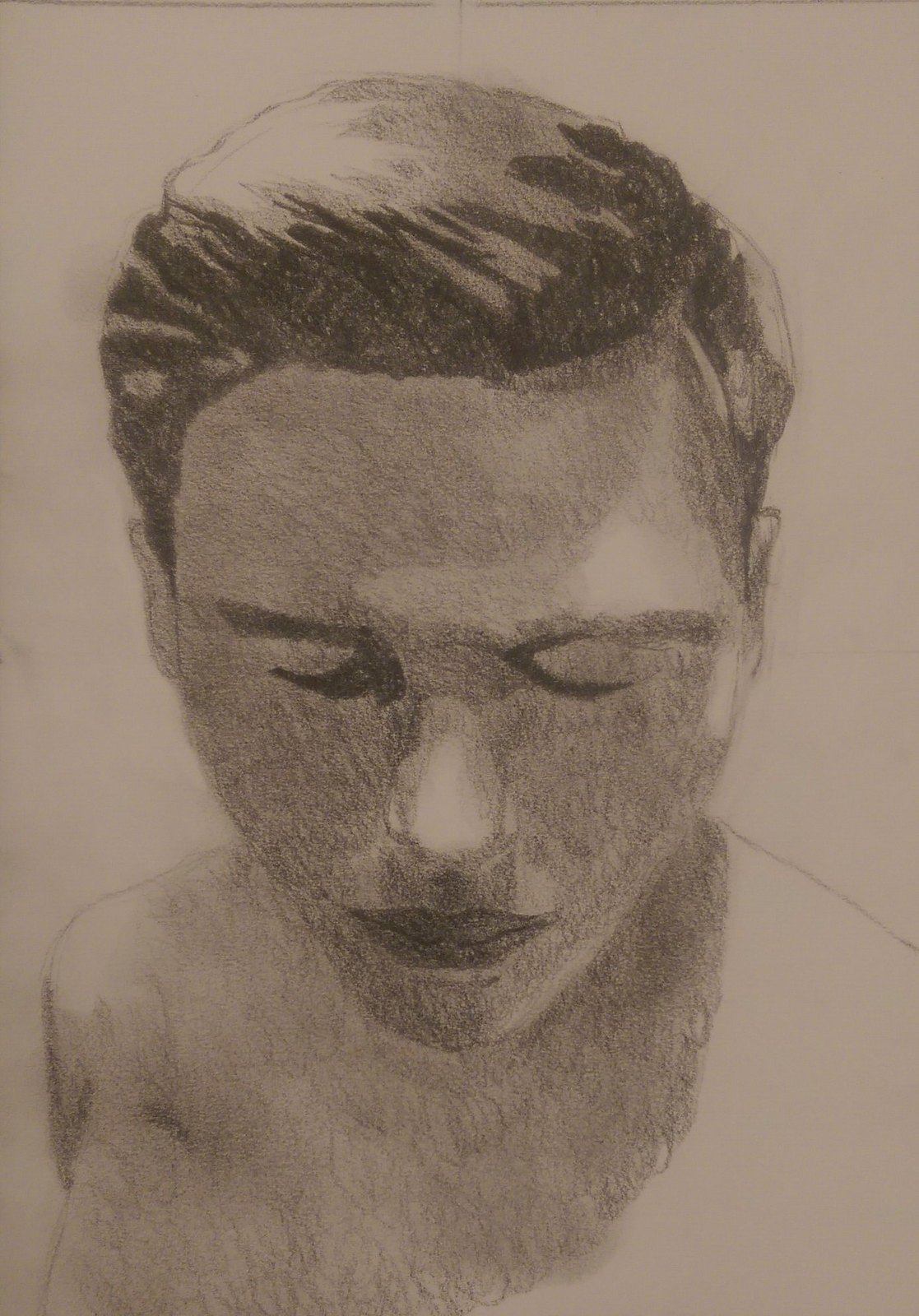A meticulously detailed pencil drawing depicts a young boy, presumably under the age of 16, on a white or light gray paper. The boy's eyes are closed, yet his face is fully oriented towards the viewer, allowing for an intricate portrayal of his facial features. Despite his closed eyes, the expression is serene and introspective. The drawing utilizes light and shadow masterfully, with illumination coming from the right side, highlighting the right side of his face and shoulder. This expert use of lighting accentuates the boy's delicate features, including a notably smaller chin and a well-defined nose, free from shadow. The overall composition is a testament to the artist's skill, capturing both the innocence and depth of the subject.